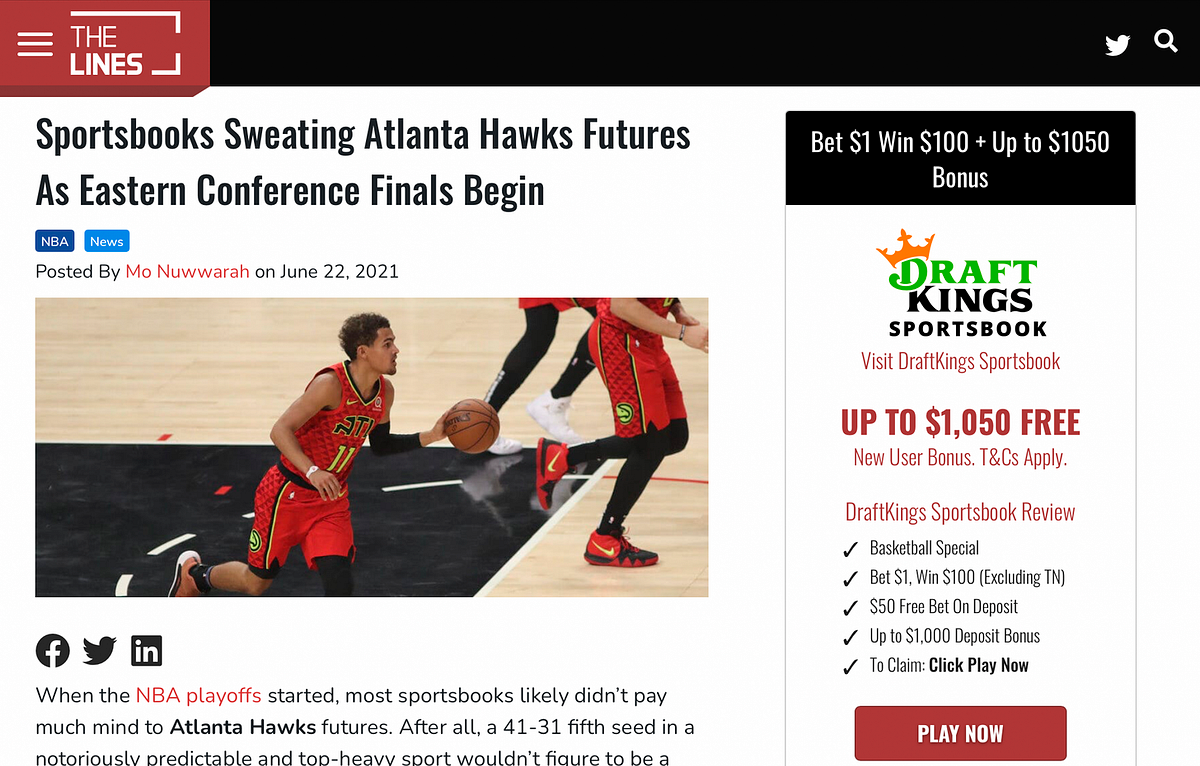At the top left corner of the image, there is a red square containing the word "LINES" spelled out in capital letters (L-I-N-E-S). Adjacent to this red square, there are three small horizontal lines stacked on top of one another. Next to this is a long black box extending to the right, featuring the iconic Twitter bird logo and a search bar.

Below this header, black text reads: "Sportsbooks sweating Atlanta Hawks futures as Eastern Conference finals begin." Beneath this text is an image of a basketball player dressed in a red and black jersey, holding a basketball and running. To the right of the player is another athlete wearing long red shorts, tall black socks, and red Nike shoes with a yellow swoosh.

Further down, black text describes the situation: "When the NBA playoffs started, most sportsbooks likely didn't pay much mind to Atlanta Hawks futures. After all, a 41-31 fifth seed in a notoriously predictable top-heavy sport wouldn't figure to beat."

On the right side of the image is an advertisement for DraftKings. The word "Draft" appears in green with an image of an orange crayon above the letter D, followed by the word "Kings." Below, in red text, it says: "Visit DraftKings sportsbook - up to $1,050 free." At the bottom of the advertisement, a red box contains the call-to-action text: "Play Now."